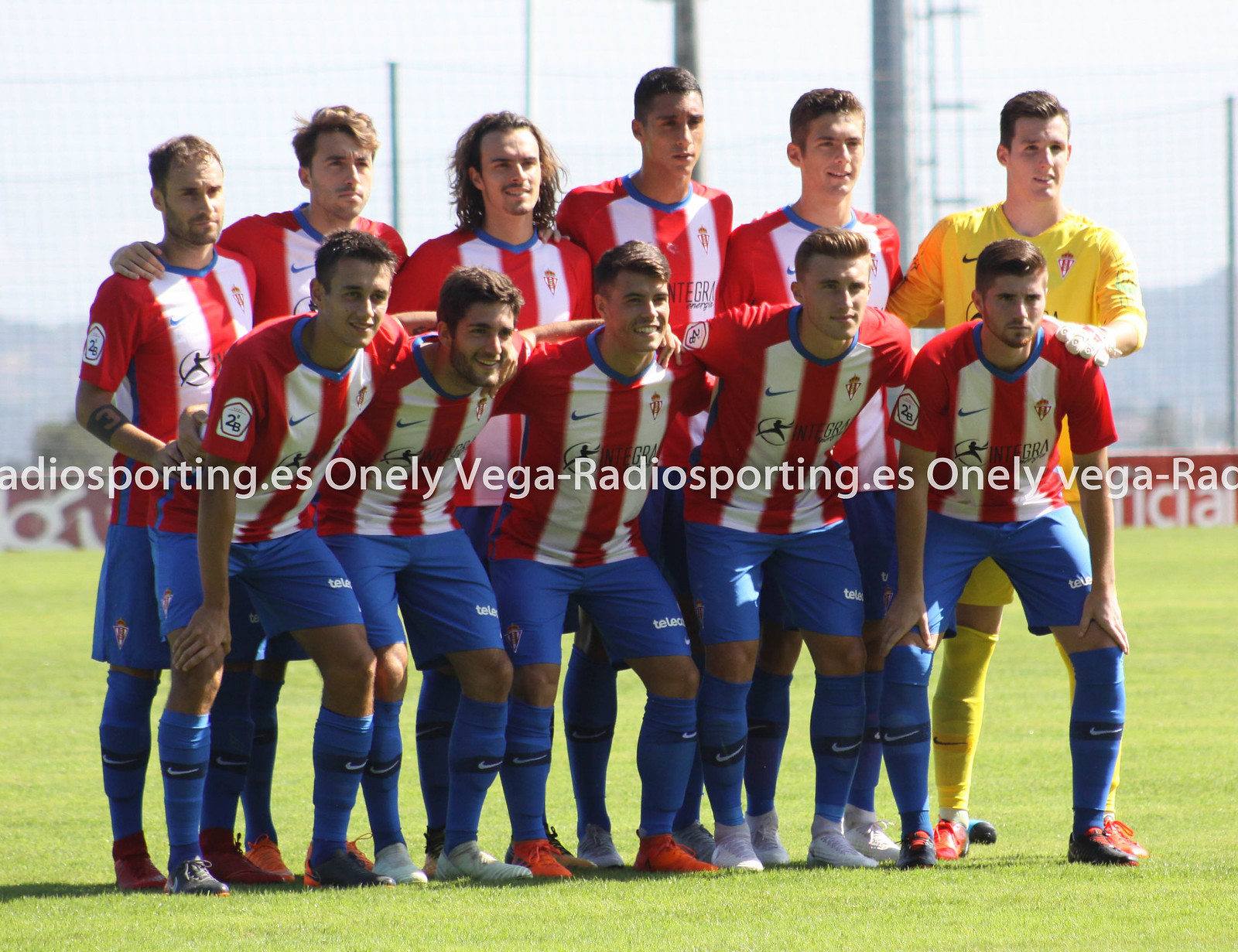This image depicts a soccer team posing for a team photo on a green soccer field. The team consists of 12 men, with 11 of them wearing red and white vertically striped jerseys, blue shorts, and tall blue socks pulled up to their knees, featuring the Nike emblem on the shins. Their footwear varies between orange, red, and white cleats. There is one player in a yellow jersey, yellow shorts, and yellow socks, likely the goalkeeper. The formation includes six men standing in the back row and five men in the front row, who are bent over at the hips, in an athletic stance. The goalkeeper is positioned between the two rows on the right side. The background shows a low wall with red and white sponsor text, possibly reading "oneleavegaradiosporting.es," though the exact wording is partially obscured. The field itself appears to have large poles for lights or power lines. The players appear to be in their early 20s.